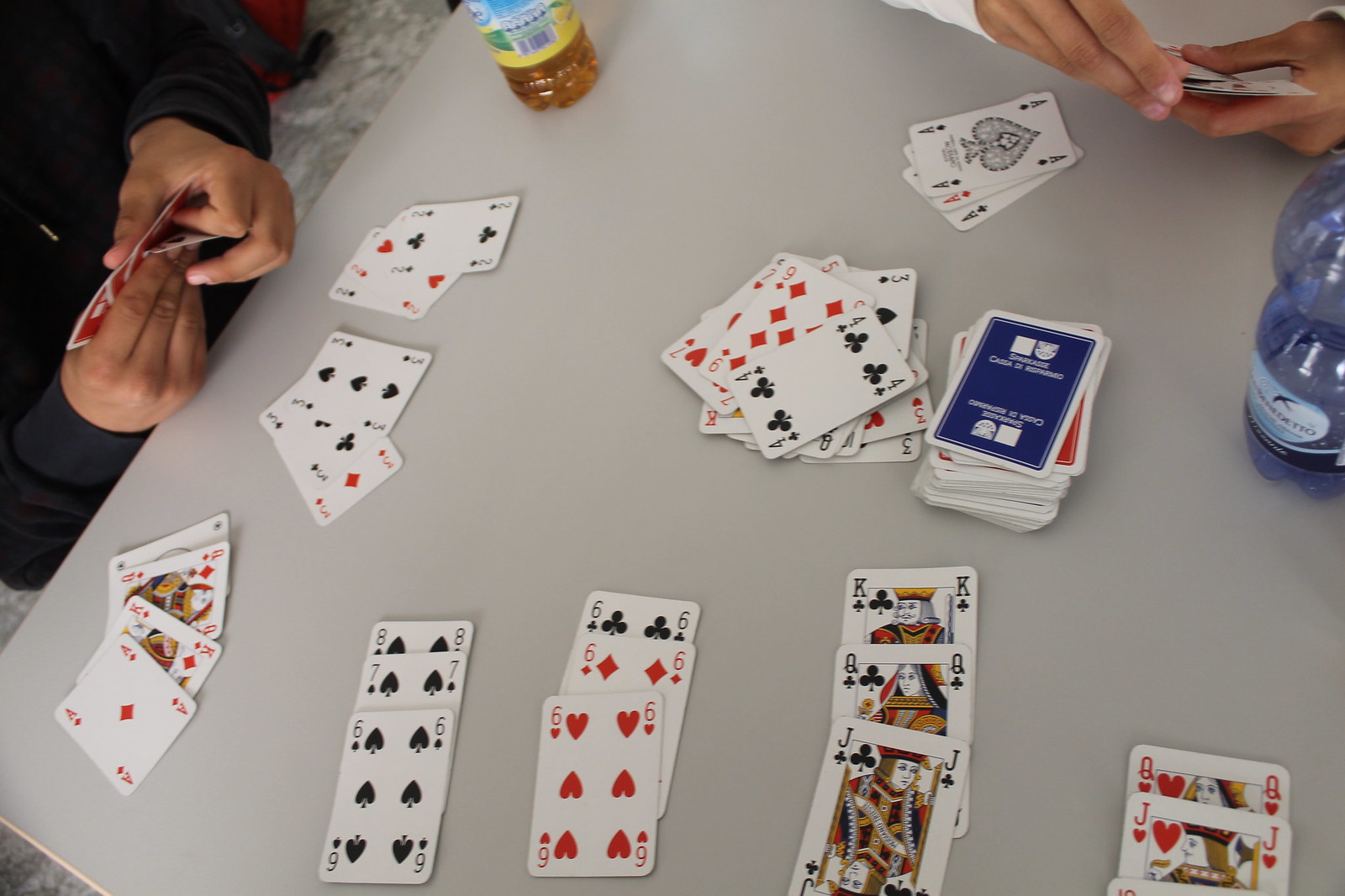In the image, two individuals are seated at a white table engaged in a playing card game. The table is scattered with a classic Solitaire deck. On the right side of the image, a person with slightly tanned skin is wearing a long-sleeved sweater. Beside him, to his left, is a transparent bottle filled with orange-gold liquid, likely a drink. This person is in the process of fanning out his cards. Adjacent to him, there's a considerable number of cards flipped over and spread out. 

On the upper left side of the table, another person with lighter skin is holding a hand full of cards and has three aces laid out neatly beside him. In the center of the table, there is a deck of cards stacked upside down, accompanied by a disordered pile of playing cards. The lower part of the table features cards organized meticulously by color, suit, and numerical order, showcasing a sequence including six to eight of clubs, three sixes from various suits, as well as a jack, a queen, and a king, with another queen and a jack belonging to different suits.